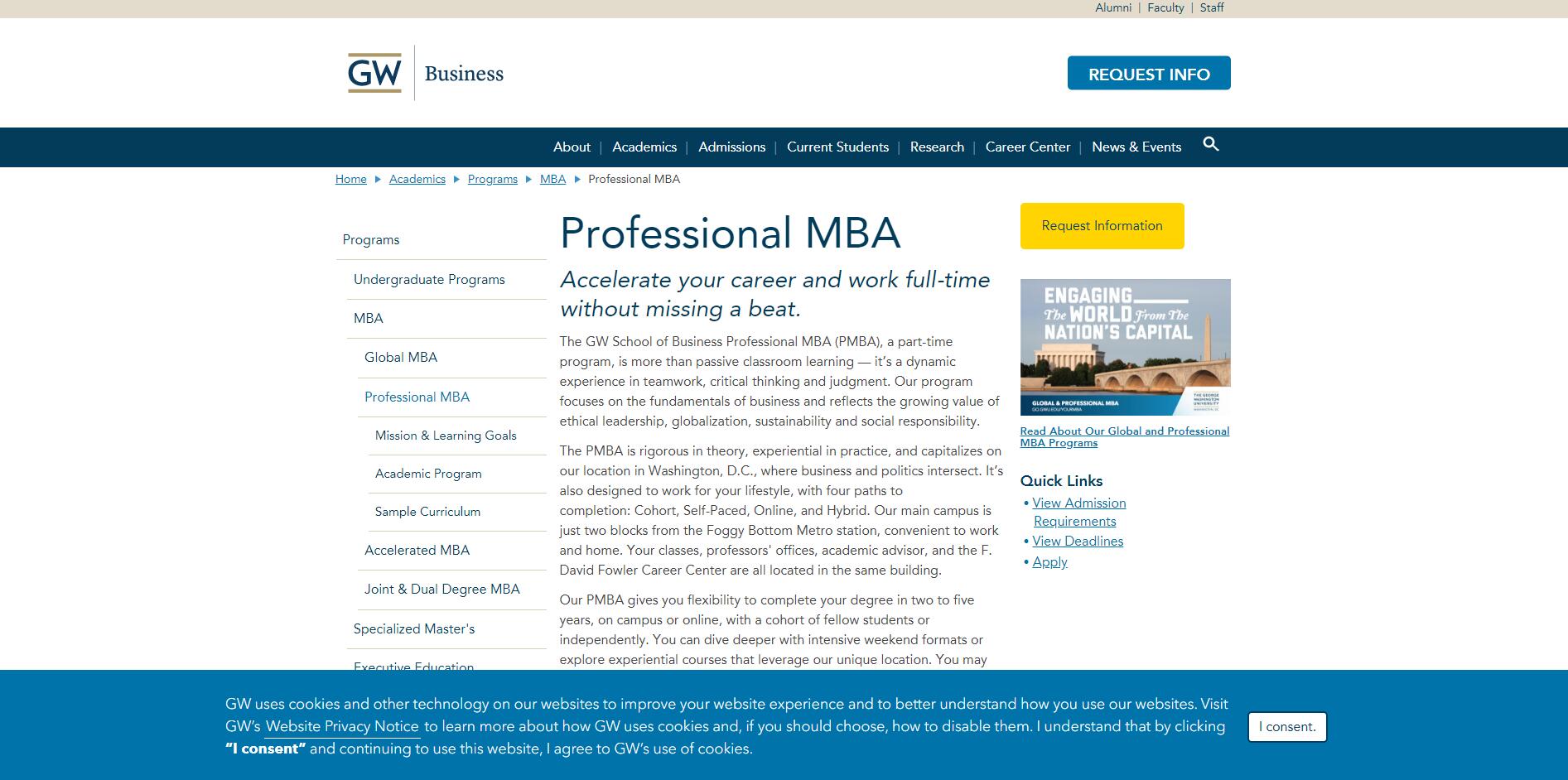This image is a cropped desktop screenshot of the George Washington University School of Business's Professional MBA informational webpage. The background is predominantly white, providing a clean and modern look. At the top left corner, the George Washington University logo is displayed prominently. To its right, the word "Business" stands out in bold blue letters. 

To the far right, a blue button labeled "REQUEST INFO" is featured, with the text in bold white capital letters. Directly below this is a horizontal blue bar that stretches across the entire page. Centered within this bar are various categories in large white font, accompanied by a search icon aligned to the far right.

The central focus of the page is the text "Professional MBA" written in large blue letters. Beneath this, the phrase "Accelerate your career and work full-time without missing a beat" is displayed in bold italicized font, capturing attention with its motivational message. Below this headline, there is detailed information about the program.

On the right side of this section, a yellow box offers another opportunity for visitors to "Request Information." Directly below the yellow box, there is a downloadable infographic or PDF file related to the MBA program. Towards the bottom right, the page features a "Quick Links" section in bold blue font, with a bullet-point list of three popular links.

Finally, at the very bottom of the page, a blue informational bar about cookies spans the width of the screen, and to the far right of this bar, a white button labeled "I CONSENT" is visible, inviting users to accept the site's cookie policy.